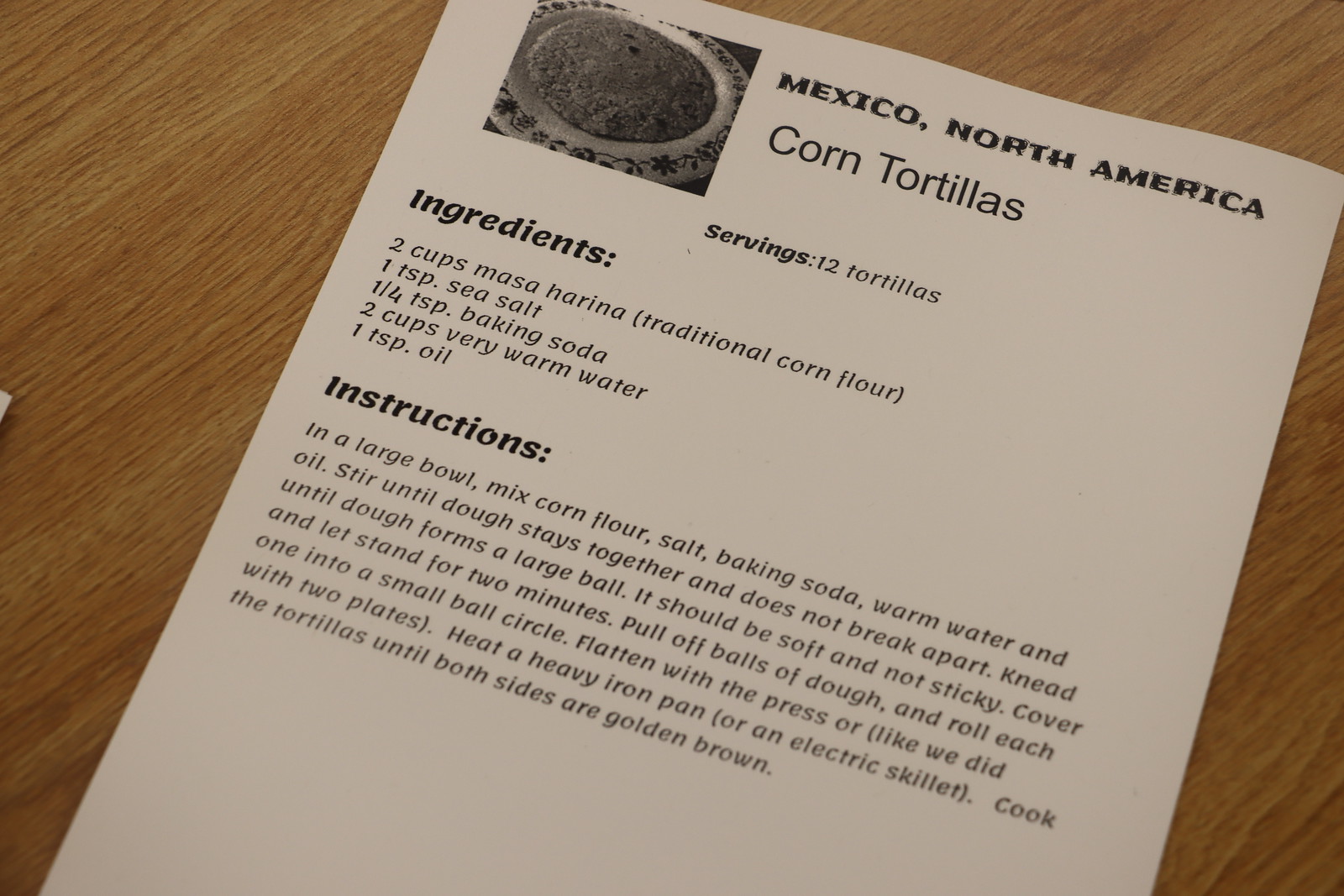The image depicts a white piece of paper laid out on an oak-colored wooden table, clearly showcasing the wood grain. The paper is a printed recipe sheet featuring a black-and-white photo of corn tortillas on a plate with a floral edge in the top corner. The header at the top of the page reads "Mexico, North America" in bold black fonts, with "corn tortillas" written in large but non-bold fonts below it. Centered under this, in smaller font, is "Serving: 12 tortillas." On the left side of the paper, a subheading "Ingredients" is listed in bold and large fonts, followed by the ingredients: 2 cups masa harina (traditional corn flour), 1 teaspoon sea salt, 1/4 teaspoon baking soda, 2 cups very warm water, and 1 teaspoon oil. Below this, another bold subheading "Instructions" outlines the preparation steps:

1. In a large bowl, mix the corn flour, salt, baking soda, warm water, and oil.
2. Stir until the dough stays together and does not break apart.
3. Knead until the dough forms a large ball, ensuring it is soft and not sticky.
4. Cover and let stand for 2 minutes.
5. Pull off portions of the dough and roll each one into a small ball.
6. Flatten with a press or use two plates to achieve a flat circle.
7. Heat a heavy cast iron pan or an electric skillet.
8. Cook the tortillas until both sides are golden brown.